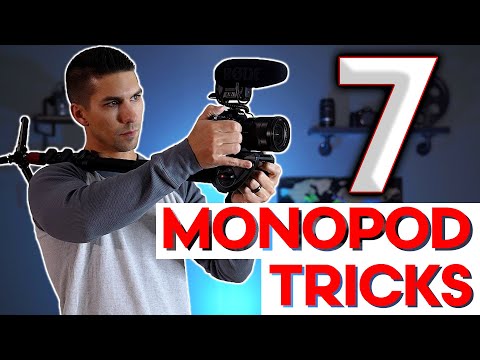The image, likely a YouTube video thumbnail, features black bars at the top and bottom framing the rectangular image. At 3 inches wide by 2 inches high, the image shows a man, seen from the torso up, standing on the left side. He has light skin, short brown hair shaved in a fade, and is wearing a long-sleeved gray shirt with a light gray torso and dark gray sleeves. The man is facing right, holding a large, presumably expensive camera with a significant attachment, possibly a microphone, over his shoulder. The camera tripod extends over his right shoulder. The man and the camera are outlined in white. To the right of him is a large number "7" in white with gray shadows, a red outline, and black shadows. Below this, in a white box with a cutout effect, the text "Monopod Tricks" is printed in black. The background features a blue wall with shelves holding various pieces of camera equipment.